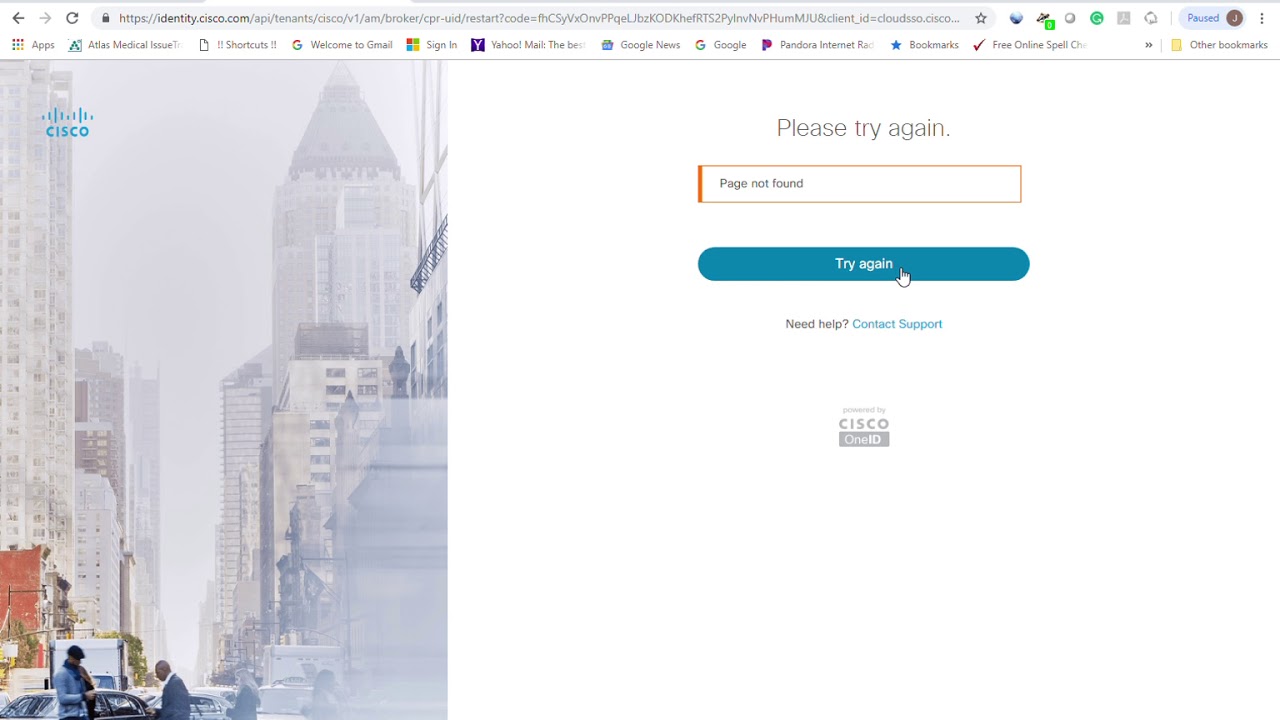The image depicts a webpage from the website identity.cisco.com. In the upper left corner, there is the word "Apps" along with an icon consisting of colorful squares arranged in a 3x3 grid, featuring red, green, blue, and yellow colors. Below this section, there is a navigation list that includes options such as "Atlantis Medical Issues," "Shortcuts," "Welcome to Gmail," "Sign in Yahoo Mail," "Google News," "Pandora Internet Radio," "Bookmarks," "Free Online Spells," and "Other Bookmarks."

A prominent identifier labeled with the letter 'J' is present, enclosed in a circular element. Additionally, a pop-up message overlaying the screen displays a "Page Not Found" error, accompanied by a prompt to "Please try again." A teal-colored rectangular button with rounded edges, labeled "Try Again," is situated within this pop-up. There is also a note offering assistance, stating "Need Help? Contact Support," with references to "Cisco One ID."

To the left section of the image, there is a photograph showcasing a city street flanked by tall buildings. In the top left corner of the photograph, the word "Cisco" appears in blue. The overall impression is that the user is experiencing difficulty accessing the page, indicated by the "Page Not Found" error message.